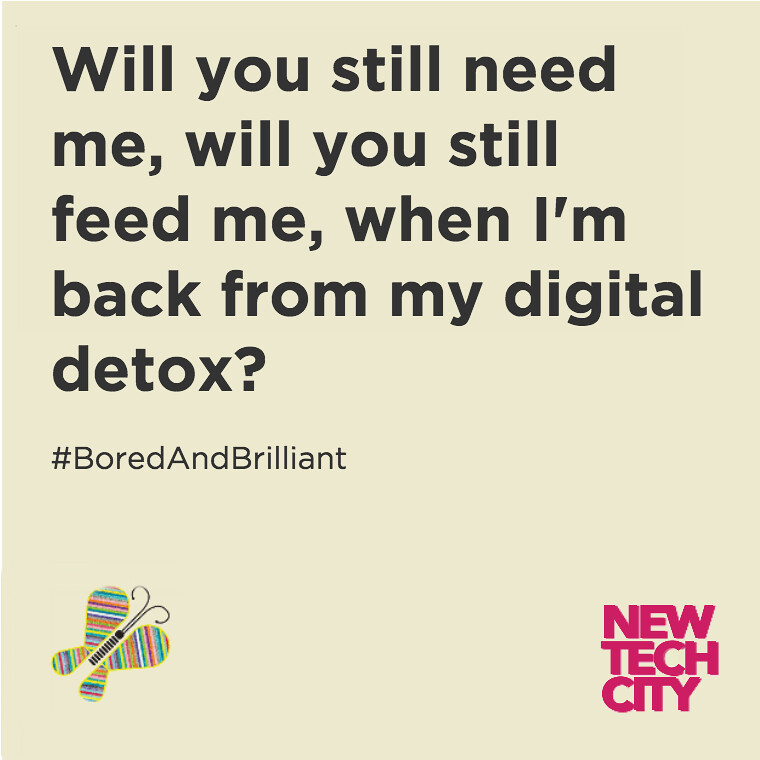The image features an ivory background with a prominent, thought-provoking quote in large black letters: "Will you still need me? Will you still feed me when I'm back from my digital detox?" Beneath this, in smaller black font, is the hashtag #boredandbrilliant. In the lower left corner, there is an artistic drawing of a butterfly adorned with random, colorful stripes, including red, yellow, green, blue, and white. To the lower right, bold capitalized letters in a bright pinkish-red color spell out "New Tech City", giving the whole composition a striking end. The layout is clean and structured, with the text centrally aligned and the butterfly and title artistically balancing each other at the bottom.